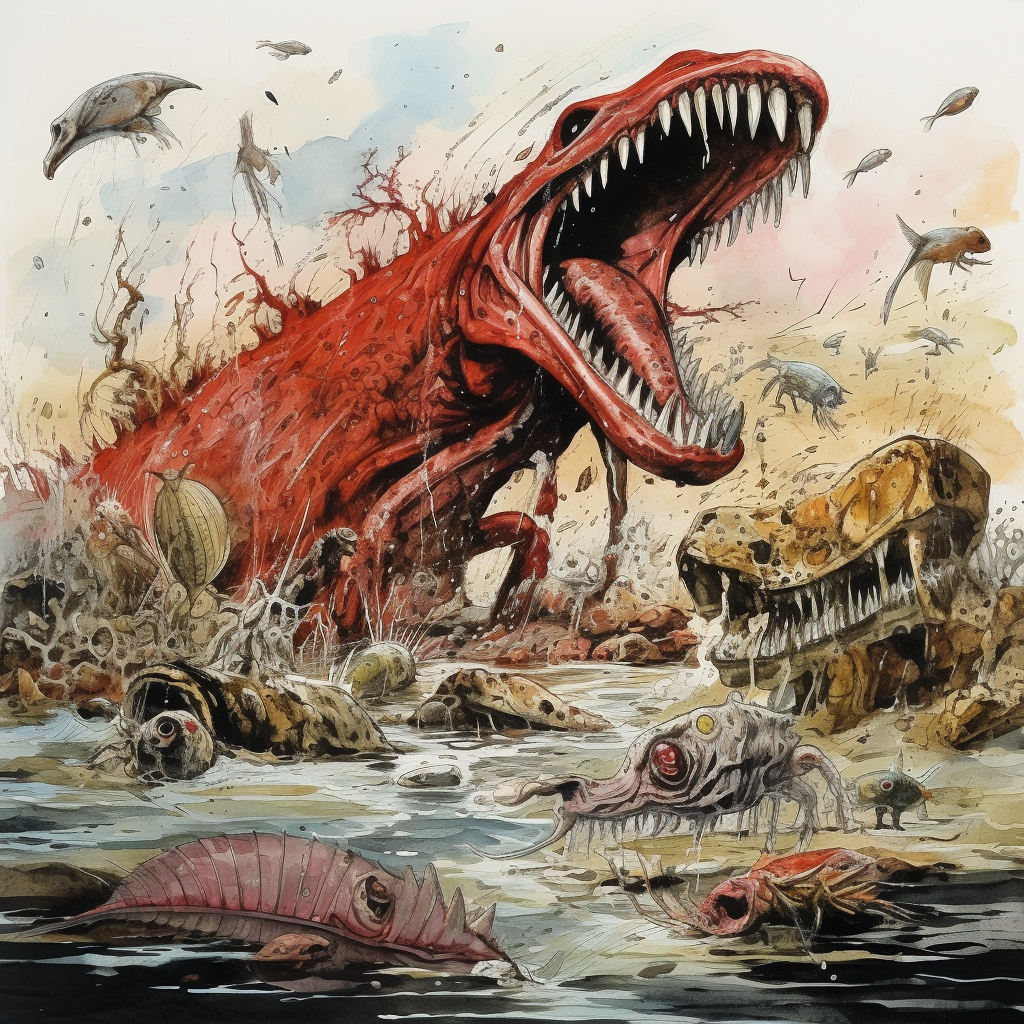The image is a detailed, square-shaped artwork approximately six inches high and six inches wide, depicting an intense underwater scene with a myriad of vivid colors and creatures. The central focus is a large, angry-looking red lizard-like monster with a long neck and body, thin arms, and additional tentacles emanating from its form. Its fierce expression is highlighted by its sharp, white teeth and a big red tongue, with its eyes being a stark white surrounded by black. The monstrous creature appears to be emerging from the ground, causing a commotion among the surrounding sea life.

To the left of the monster, the foreground features a series of bones or exoskeleton casings with dead fish bodies among other fish floating nearby. Various unusual creatures resembling a mix of tadpoles and other forms are scattered throughout the scene. Additionally, a pink-colored creature, resembling a slug, is positioned in the lower left corner.

On the right side, the image showcases more bizarre sea creatures, including a combination of orange, pink, and yellow cricket-like beings and a white blobfish. Among them, there is a peculiar treasure chest with a cow face on its exterior and filled with sharp teeth lining the inside. In the background, colors range from white, blue, red, tan, to light brown, lending depth and vibrancy to the chaotic underwater environment. Small flying crabs and manta-like fish add to the sense of disorder as they navigate through the air above the fray. This rich illustration captures a scene reminiscent of a fantastical sea creature battle, filled with dynamic and grotesque details.